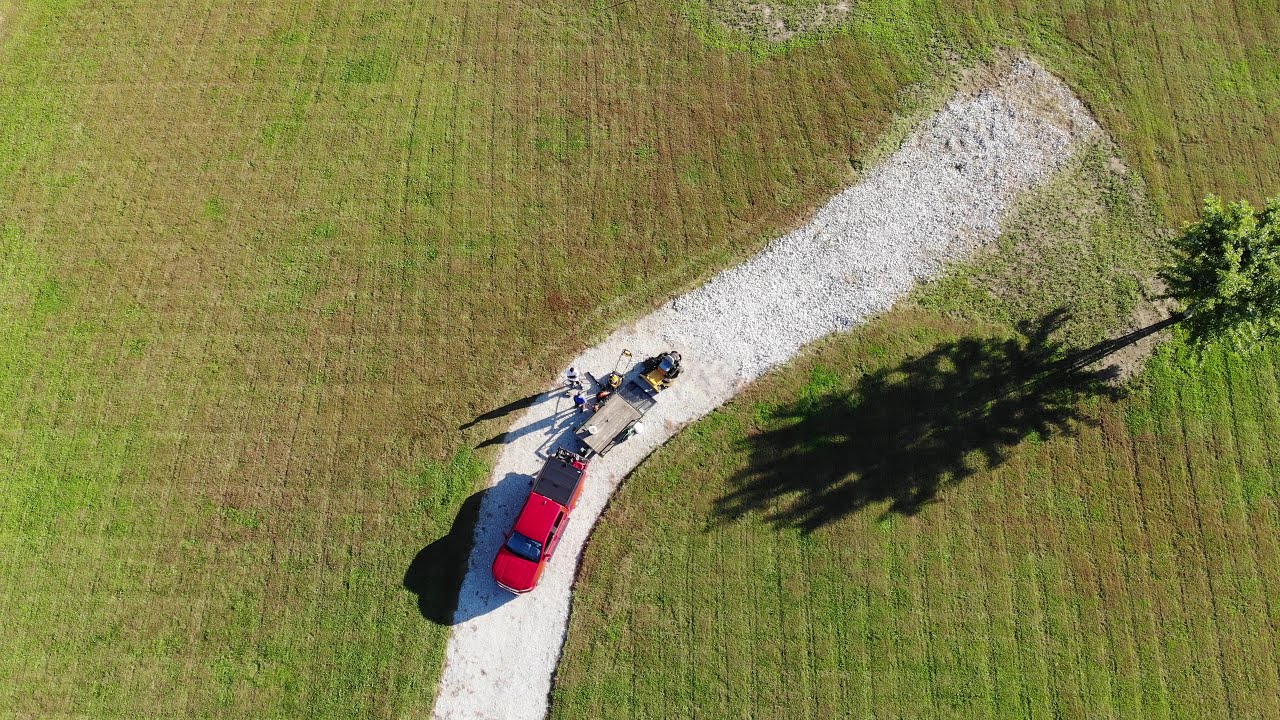This detailed aerial photograph, likely taken from a drone or aircraft a couple hundred feet up, captures an expansive grassy field. The field is primarily brown, indicating possible water deficiency, with patches of green and a distinct crisscrossed grid pattern suggesting recent mowing, especially evident on the right side. Toward the right edge of the photo, a slender deciduous tree, not very old, stands out, casting a long shadow to the left under the bright sunlight.

Dominating the center of the image is a gray gravel road, about two lanes wide, that arcs to the right and culminates in a broader gravel area. Parked on this road is a red pickup truck, viewed from above, with a trailer hitched to its rear. The trailer contains a small green tractor with a yellow bucket and a riding lawnmower, possibly reflecting a landscaper's equipment. Additionally, a push lawnmower is visible nearby.

Indicating human activity, several figures can be seen around the truck, their shadows elongating on the gravel road and adjacent field. The overall scene suggests a recently completed landscaping job, underscored by the orderly mowed patterns in the field and the presence of the lawn maintenance equipment.